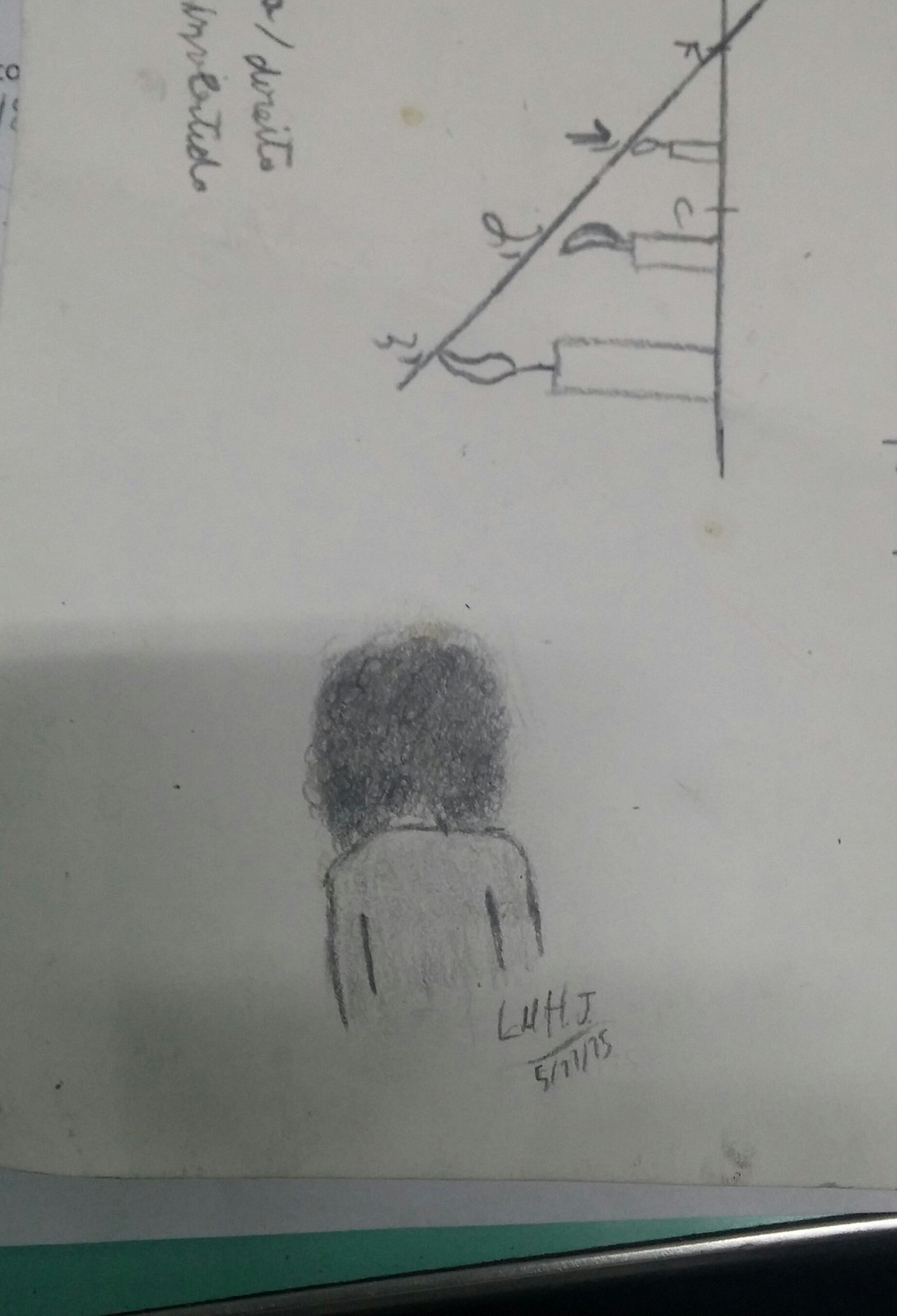This photograph captures a detailed pencil sketch on white printer paper, positioned on what appears to be a metal tray likely placed on a desk. Dominating the lower section of the sketch is a figure, possibly a man or woman, characterized by long, curly hair and a long-sleeved shirt. The figure faces away, obscuring any other facial features or details. Below this figure are the initials "L-H-H-J" and a date that seems to read "5-23-75." A shadow casts across the bottom edge, suggesting the presence of a light source nearby.

Moving up the sketch, there's a small graph-like illustration tilted to the left. This graph features three candles of varying heights, each topped with a flame. Intriguingly, a line has been drawn through these flames, though its significance is unclear. To the upper left side of the sketch, there's some cursive writing, which is difficult to decipher. The entire composition is rendered in black and white, with meticulous pencil strokes capturing the details of both the person and the accompanying symbols.